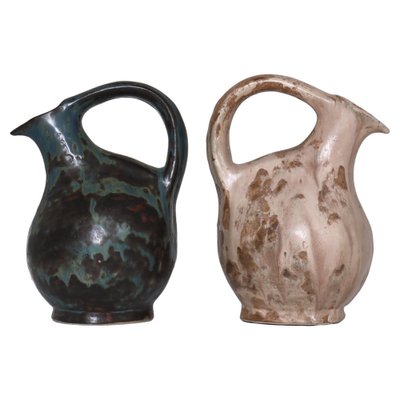This image depicts two identical clay jugs or pitchers, positioned facing away from each other against a stark white background, as if they were back-to-back. Each jug features a prominent handle located higher up and a small spout angled to the side, creating a mirrored effect between the two vessels. They both have a round, spherical body and a sturdy flat base.

The pitcher on the left is primarily a dark green color with accents of black, brown, and faint red, displaying a mottled pattern that gives it an aged, almost excavated appearance. Its counterpart on the right is predominantly beige, embellished with darker brown and red splotches, conveying a sense of weathered antiquity. Both jugs share a smooth texture but exhibit a splotchy design in their coloring, contributing to their decorative charm. Their handles connect the top openings to the rounded bases, highlighting their unique, almost artifact-like quality.